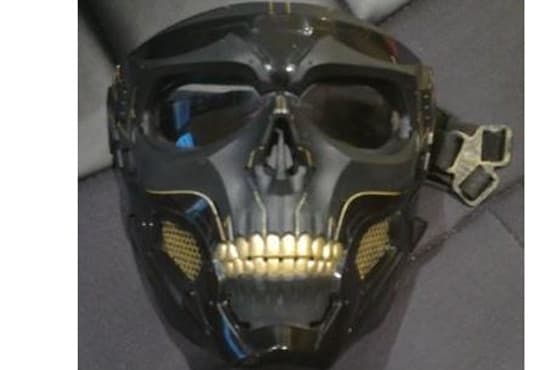This image depicts a detailed, black skull mask designed to cover the entire face, suitable for use as a Halloween costume or possibly as part of a helmet. The mask is crafted from a material that appears to be plastic and features a strap with metal buckles for securing it over the head. The eye sections are covered with clear plexiglass, allowing visibility while worn. Notably, the mask includes gold-colored teeth in the front and breathable mesh venting on both sides of the cheeks for air circulation. The image is taken indoors on a soft, dark gray surface, enhancing the dramatic appearance of the mask.